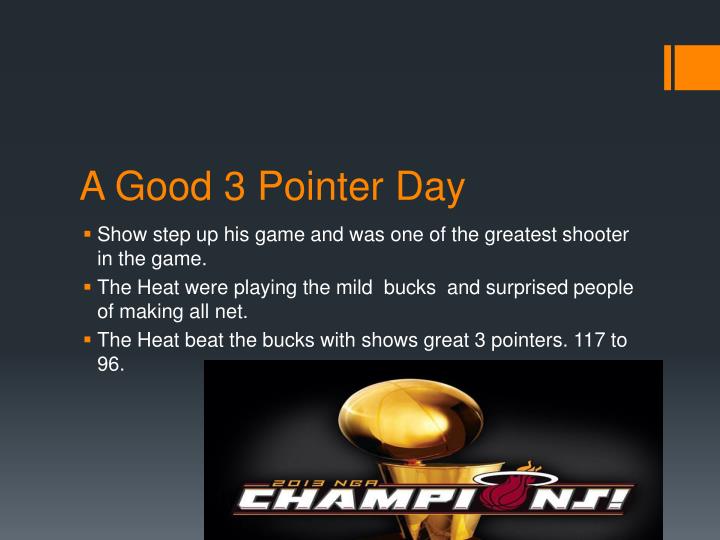The poster is a horizontal rectangle featuring a dark gray background that fades to a lighter gray towards the bottom. Just above the center and left-aligned in orange text, the title reads "A Good Three-Pointer Day." Beneath the title are three orange square bullet points with white text. 

The first bullet point states, "Show stepped up his game and was one of the greatest shooters in the game." The second bullet point reads, "The Heat were playing the Mild Bucks and surprised people by making all net." The final bullet point says, "The Heat beat the Bucks with Show's great three-pointers, 117 to 96."

At the bottom of the poster is a black horizontal rectangle that fades to a lighter gray at the center. Within this rectangle is an image of a gold basketball trophy. Across the trophy, in white uppercase letters, is the word "CHAMPIONS," with the "I" in "CHAMPIONS" stylized as a red basketball with a white ring around it. Just above, in smaller gold text, it says "2013 NBA."